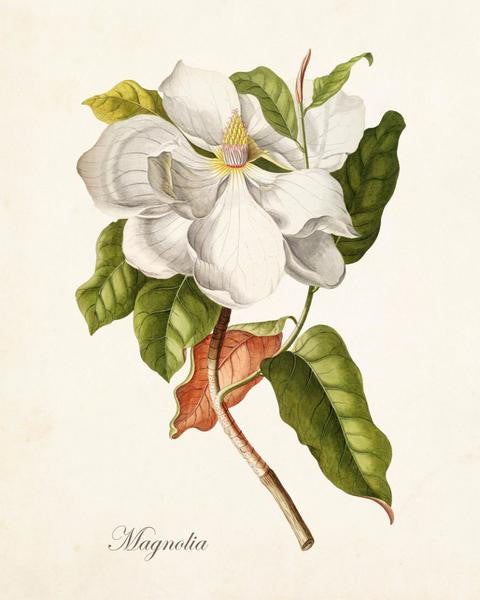This detailed up-close scientific drawing, an artistic rendering of a fully bloomed magnolia blossom, is set against a white parchment paper background. The magnolia, labeled "Magnolia" in cursive in the bottom left corner, features elegant, white petals encircling a central cluster of pistils that are yellowish with some white at the base, indicating pollen. The large blossom dominates the center of the image, with several green leaves attached to an earthy, rich brown woody stem that is cleanly cut at the bottom. Notably, some of the leaves are folded inward, revealing a brown-red hue underneath. This precise illustration showcases the beauty and detail of the magnolia, meticulously resting on the light tan, parchment-like surface, inviting close observation.